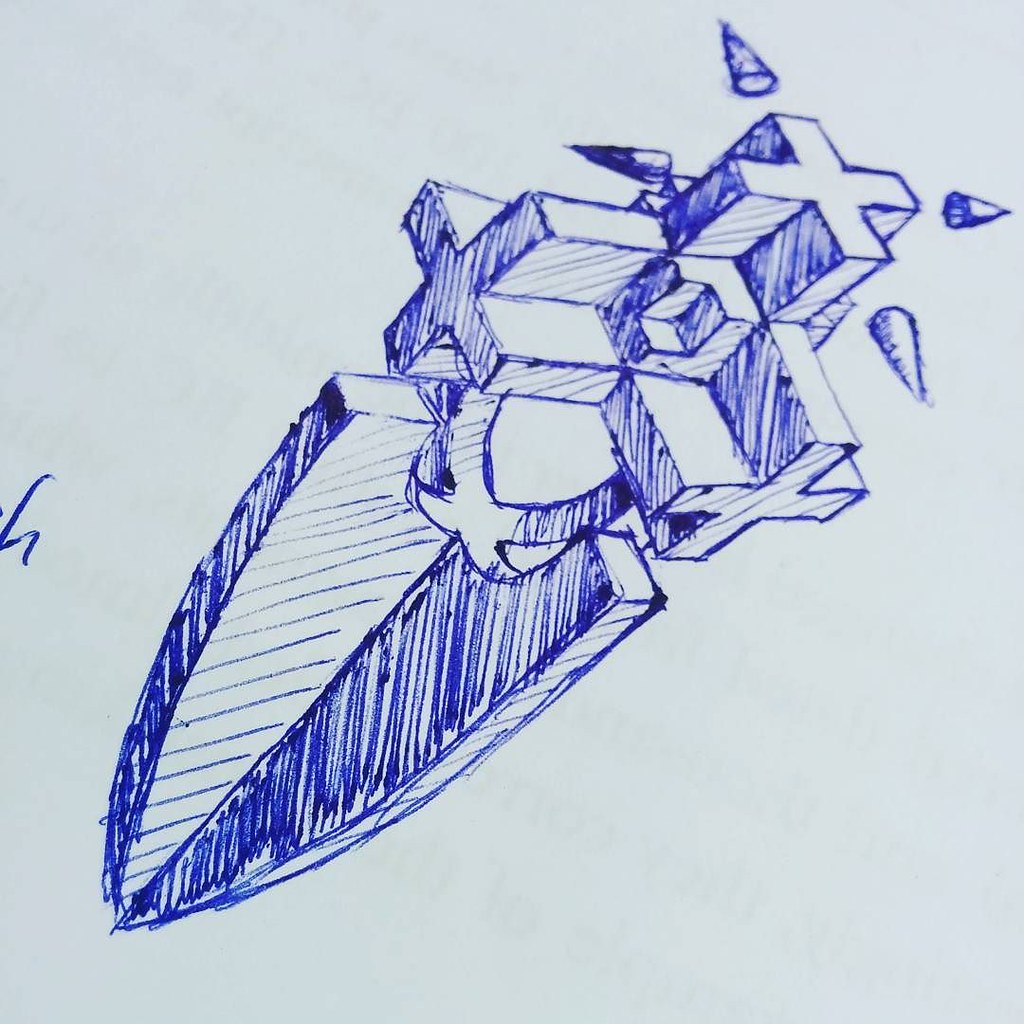This photograph captures a detailed sketch drawn in blue ink on a light gray background. The central focus of the drawing depicts a 3D geometric structure with a thick base that resembles an armor-piercing dagger or a shield, culminating in a pointed, arrow-like tip at the bottom. The handle of this structure is intricately designed, featuring a central cube from which cross-shaped prisms or large plus-signs extend outward in an X pattern. The sketch appears to progress diagonally from the bottom left, where two tall, building-like towers are drawn and shaded in dark blue, creating a sense of depth. As the eye moves upward, more complex shapes emerge, including additional 3D cubes and cone-like objects that give the entire form a dynamic and layered appearance. The entire composition, meticulously rendered in blue ink, conveys a fusion of architectural precision and creative abstraction.